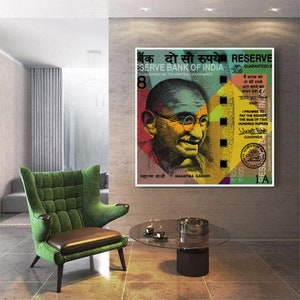The photograph depicts an indoor setting with a brown tile floor. Centrally located on the wall is a large poster featuring a portrait of Mahatma Gandhi, with glasses and text that reads "Serve Bank of India Reserve," in varying colors from yellow to orange to green. Next to the wall, positioned to the left, is a green velvet chair with brown accents, a wide cushiony back, and long, slender brown legs. The seat of the chair has an indistinct object lying on it. Adjacent to the chair on the right is a glass oval coffee table, which appears to be mounted on a stand reminiscent of an old cylindrical ashtray. On the table are two silver chrome cups with steam rising from them, placed on saucers. The background extends to another room with white walls and curtains, completing the cozy, possibly office-like, ambiance of the scene.